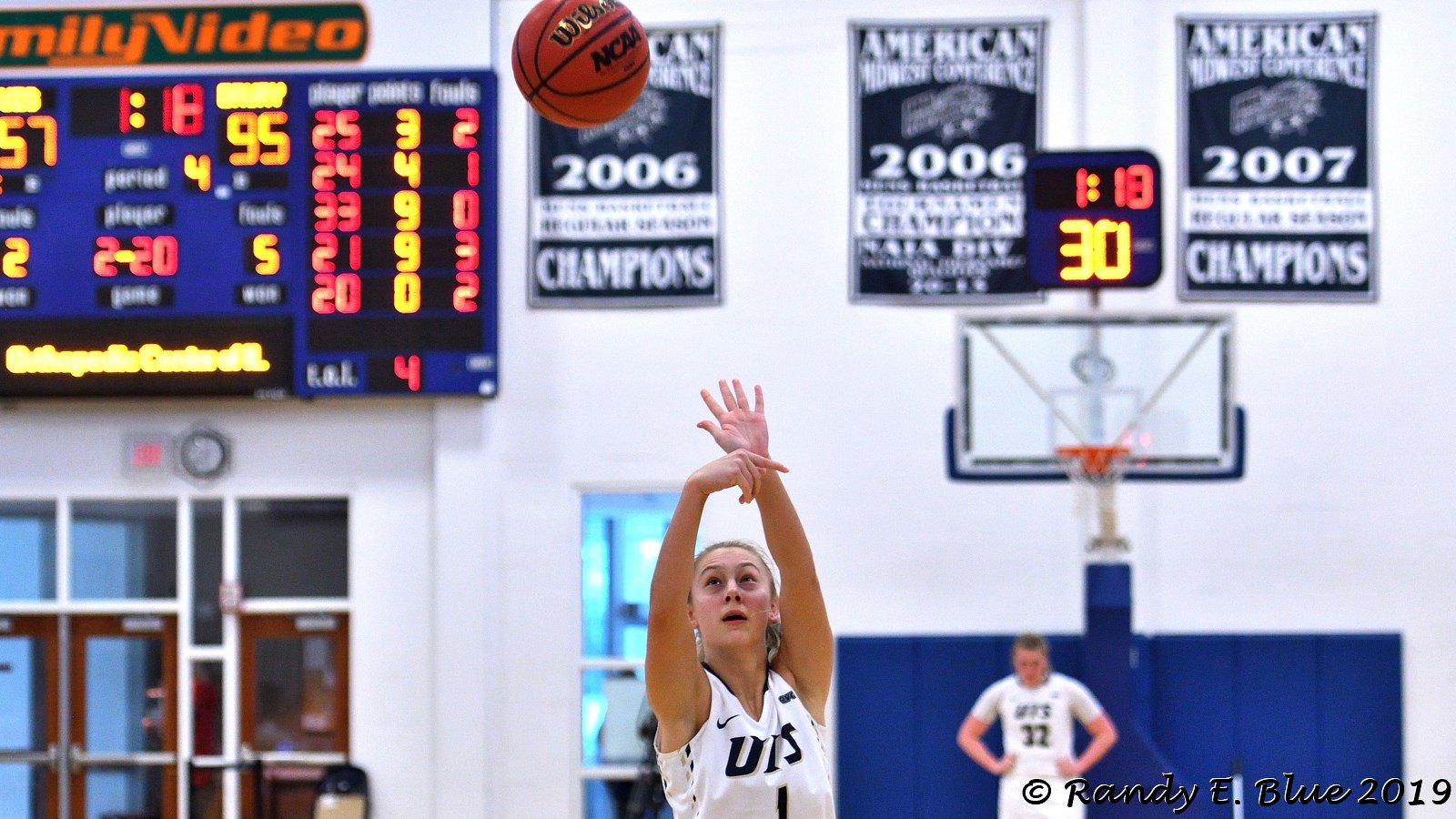The photograph captures a dynamic moment in a basketball game set inside a gymnasium. Central to the image is a Caucasian girl basketball player with blonde hair, wearing a white sleeveless jersey bearing dark navy blue letters that appear to form the abbreviation "UIS." She is captured mid-action, having just thrown a basketball that is seen at the top edge of the frame, almost cut off. Her right hand is curved in a precise follow-through motion while her left hand, fully extended, supports her throw. Her fingers are splayed as if ensuring the perfect trajectory of the ball.

In the background behind her, another player from the same team is visible, wearing a similar white uniform, marked with the number 32. This player's figure is slightly blurred as she looks downward, positioned near the far-end backboard and basketball hoop. The backboard features a blue bottom with the remainder in white.

Prominently displayed on the back wall of the gym are several banners and a scoreboard. The scoreboard, located on the upper left side of the image, has a blue background with yellow and red digits indicating the game’s statistics, though details are unclear. Above this scoreboard, an advertisement for "Family Video" is partially visible. Adjacent to the scoreboard are three black championship banners with white text and graphics. The banners commemorate past victories, specifically detailing the years 2006 and 2007 as championship years. Towards the bottom of the frame, directly below the large scoreboard, doors and a clock are faintly visible, adding to the context of a well-attended sporting event. The overall scene emphasizes the action and spirit of the game, spotlighting the athlete's focused determination as she propels the basketball mid-air.